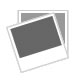The aerial image reveals a large in-ground swimming pool with a unique layout, characterized by a light green strip and a darker green interior at one end. Adjacent to the pool on the right is a crescent-shaped building, possibly housing changing rooms or amenities. This building stretches along the pool's length, accompanied by a long rectangular light green strip featuring a dark green layer within it. To the left of the main pool, there is a smaller, round area, likely a hot tub or jacuzzi, possibly covered and surrounded by numerous lounge chairs.

On the far right side of the image, there is a sizable parking lot with various cars, predominantly white, including long 70s or 80s-style vehicles and a distinctive old-school white Beetle. The parking area extends further right with a noticeable arrangement of cars, including four on one side and two on the other, with additional cars further along.

The left-hand side of the image suggests a sprawling golf course, identifiable by its rolling greens, half-circle, and oblong sand traps within the grass. The area also features a smaller parking lot and a few more buildings, indicating a well-established facility, potentially a resort or a community center. In the background, there is a glimpse of a body of water and a scattering of trees, providing a serene backdrop to the scene.